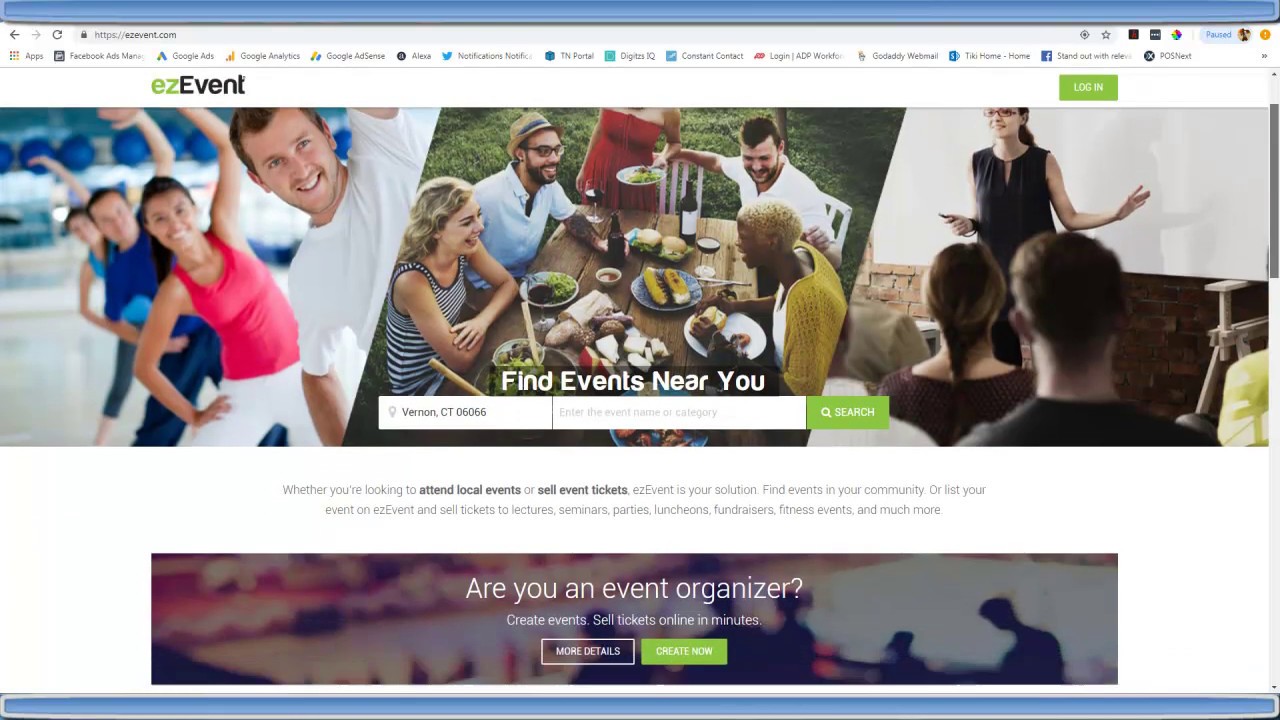On the Easy Event website, located in the upper left-hand corner, the text "Easy" is presented in a green font, while "Event" appears in black. To the far right of the page, a green "Login" button is visible. Dominating the top half of the website is a row of three side-by-side photographs. The first image depicts a group of people participating in an exercise class. The central photograph captures four individuals sitting at a picnic table, enjoying a meal and laughing together. The third image on the right shows a group seated in chairs, attentively watching an instructor standing near a whiteboard.

Beneath these images, at the bottom middle section, there is a prominent "Find Events Near You" section. This includes two fields intended for user input: one for entering the location details, such as city, state, and zip code, and a green "Search" button to initiate the search.

Continuing further down the page, another photograph is displayed. Overlaid on this image is a text in white font that reads, "Are you an event organizer?" Below the text are two buttons: one labeled "More Details" and another green button with text that is not legible due to the small screen size.